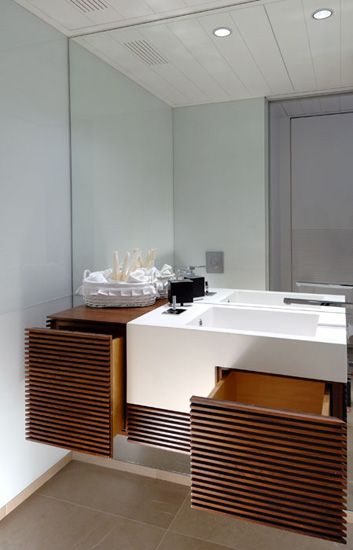This image captures a sleek, contemporary bathroom characterized by its modern design elements. The space is illuminated by recessed ceiling lighting, featuring two small lights and what appears to be a discreet heater or fan unit. The bathroom door showcases a medium gray hue, while the walls are painted in crisp white, enhancing the modern aesthetic.

A notable feature is the sophisticated vanity area, which includes a large sink with a stylish faucet. The vanity unit has two spacious drawers, both partially open, showcasing their ample storage capacity. The drawers are adorned with a textured wood finish, featuring intricate ridges that add a touch of elegance to the design. Below the sink, there's a similarly ridged area that complements the drawer design.

On the left side of the sink, a compact counter holds a container with toothbrushes, adding a functional touch to the contemporary setting. Overall, the bathroom exudes a modern charm with its thoughtful design and detailed finishes.